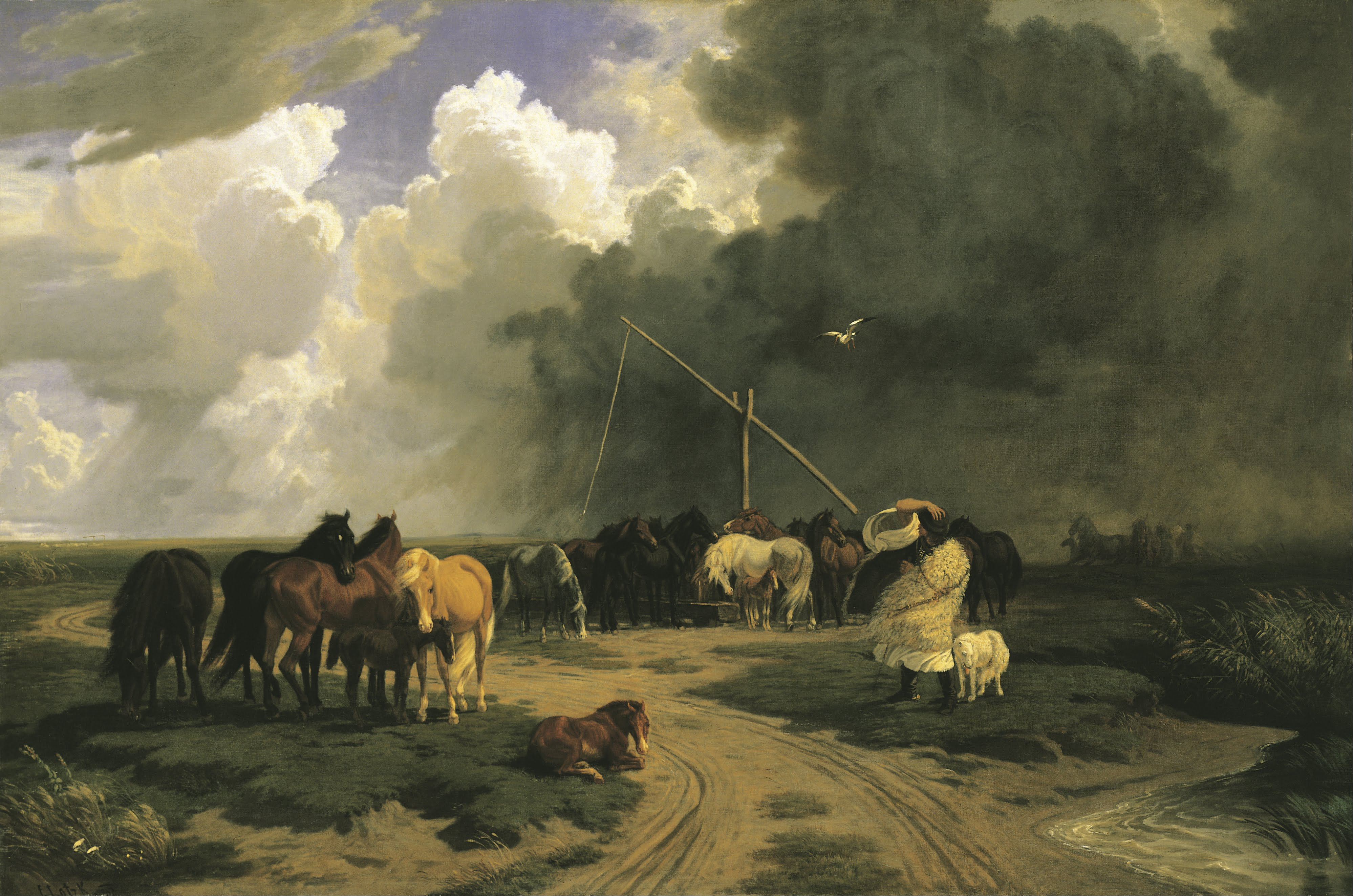This horizontally aligned rectangular painting vividly depicts a pastoral scene under a dramatic sky. The upper half showcases a sky with various types of clouds: white fluffy ones tinged with blue occupy the left, transitioning to darker, smoky clouds with a hint of gray smoothing out towards the center and right. The lower half features a landscape split by a dirt trail flanked by patches of grass. Traces of a carriage are visible on the dirt path. On the left, among the lush grass, a light brown horse lies down while three dark brown horses and a light brown one stand nearby. Dominating the center of the painting is a group of diverse-colored horses, including gray, white, and several shades of brown, possibly gathered around a hidden watering hole. To the right, a heavyset woman in a dress, coat, and hat stands with her back to the viewer, accompanied by a small white lamb. The background features additional shrubbery and a hint of a tree patch, contributing to the secluded, rustic atmosphere. The overall scene suggests a serene yet bustling countryside, possibly under the watchful gaze of an unseen herdsman. The earthy tones are complemented by dashes of green, yellow, tan, and other natural colors, all contributing to an inviting, immersive visual experience typical of evocative museum pieces.